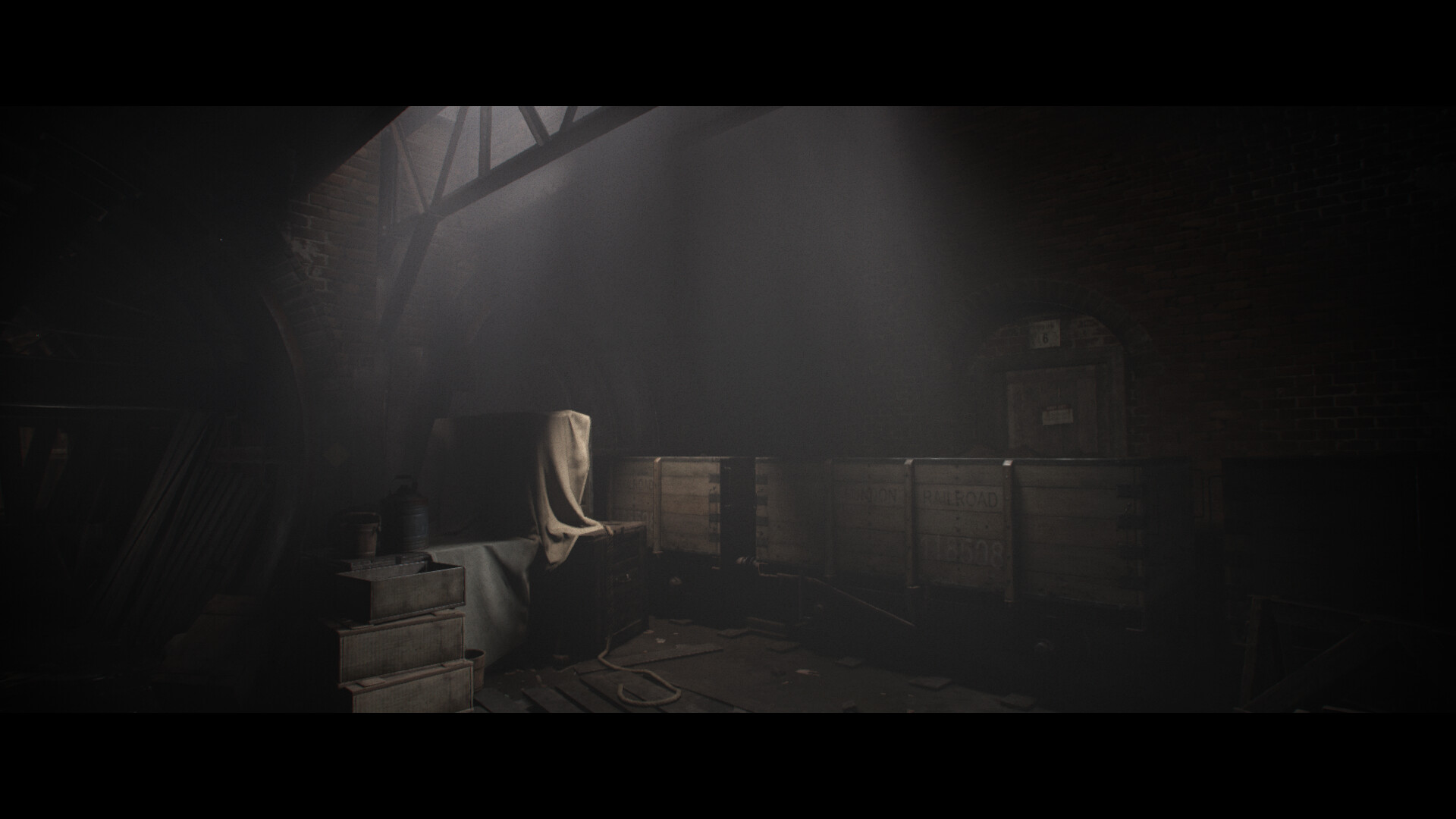This image depicts a 3D rendering of a dimly-lit, abandoned railcar station with a distinct 16:9 aspect ratio, framed by black borders at the top and bottom. The scene is quite dark, though there is some sunlight streaming in from the top, illuminating parts of the room. 

In the foreground on the left, there are three stacked metal crates and a cluster of poles situated in a rounded, tunnel-like area. Scattered across the floor are various items, including rope. The room contains an array of wooden crates and boxes, some covered in lighter-colored cloth, giving the space a disheveled appearance. 

Amidst the clutter, a rusty old lifting winch can be spotted, and metal beams stretch across the ceiling, adding to the industrial ambiance. Along the back wall, partially obscured by shadows, stand several railroad cars or mining carts. The far end of the room appears to have a concreted-over exit, contributing to the abandoned and isolated feel of the scene.